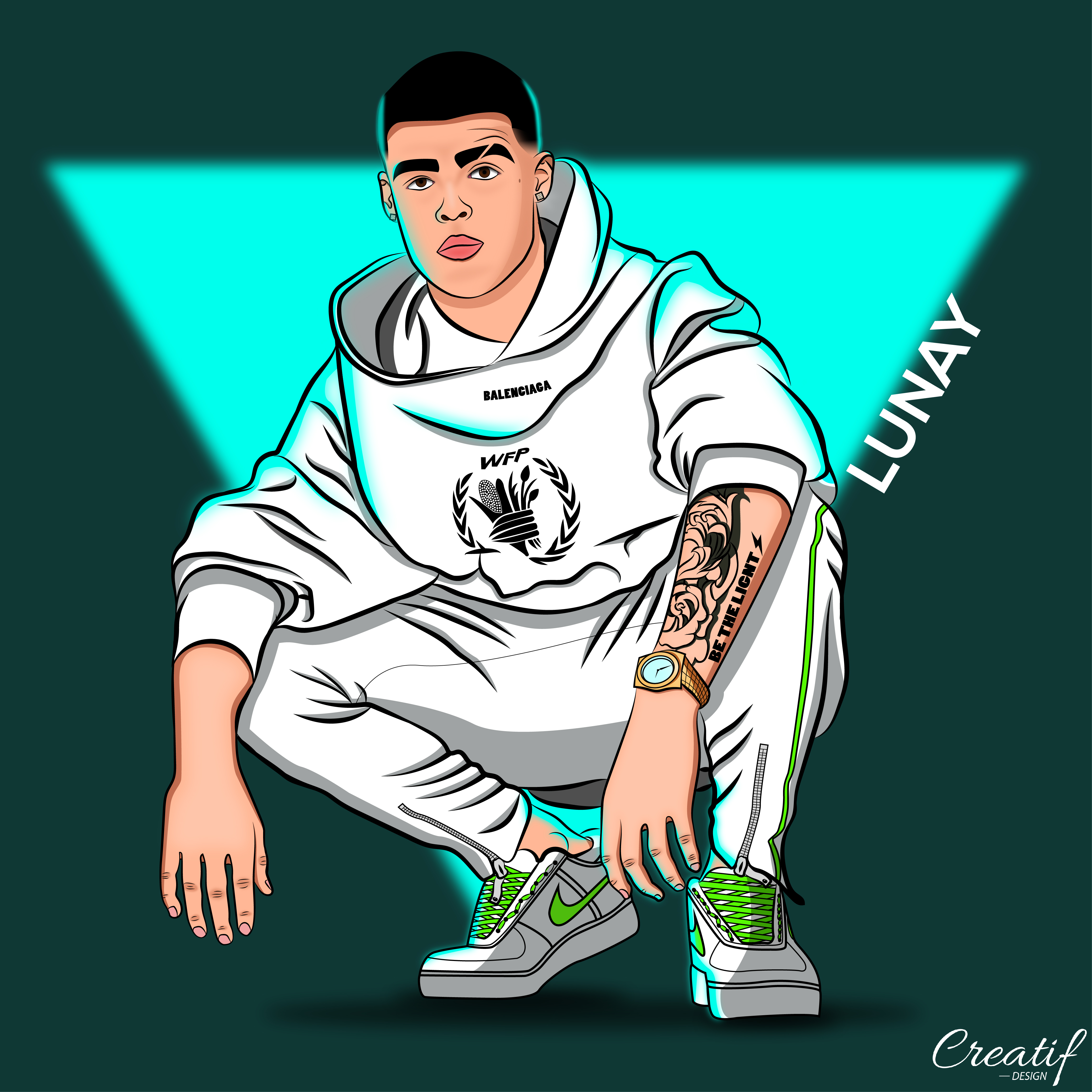This is a detailed cartoon drawing of a man, possibly a soccer player, set against a dark emerald green background with an upside-down aqua-colored triangle in the center. To the right of the triangle, the name "Lunay" is written in white lettering. The man is depicted crouching in a white tracksuit that has a black circular logo with "WFP" printed on the front, along with floral and arrow-like designs. The tracksuit features a yellowish-green line running up the side, and the hood bears the word "Balenciaga." 

He is wearing white Nike shoes with neon green laces and a matching neon green swoosh. On his left wrist, he sports a gold watch with a blue face and has a black tattoo on the same arm that reads "be the light" alongside a lightning bolt and some wavy patterns. His black hair is styled short with a line shaved into his left eyebrow. He also has earrings in both ears. In the bottom corner of the image, the words "creative design" are inscribed, adding an additional layer of detail to the artwork.